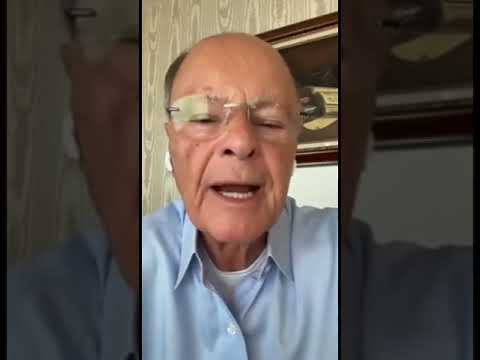In the center of the image is an elderly man, likely in his 60s or 70s, who is almost bald with a few strands of brown-grey hair on the right side of his head. He is wearing clear glasses and white earphones, and he is dressed in a blue collared button-down shirt with visible clear buttons, over a white t-shirt. His mouth is open, showing his lower teeth, suggesting he is speaking, possibly into a phone as he stares downward. The background features beige wallpaper with a darker beige and white oval pattern on the left side, transitioning to a wood grain paneling on the right. There is also a mounted artwork in a brown frame on the wall behind him.